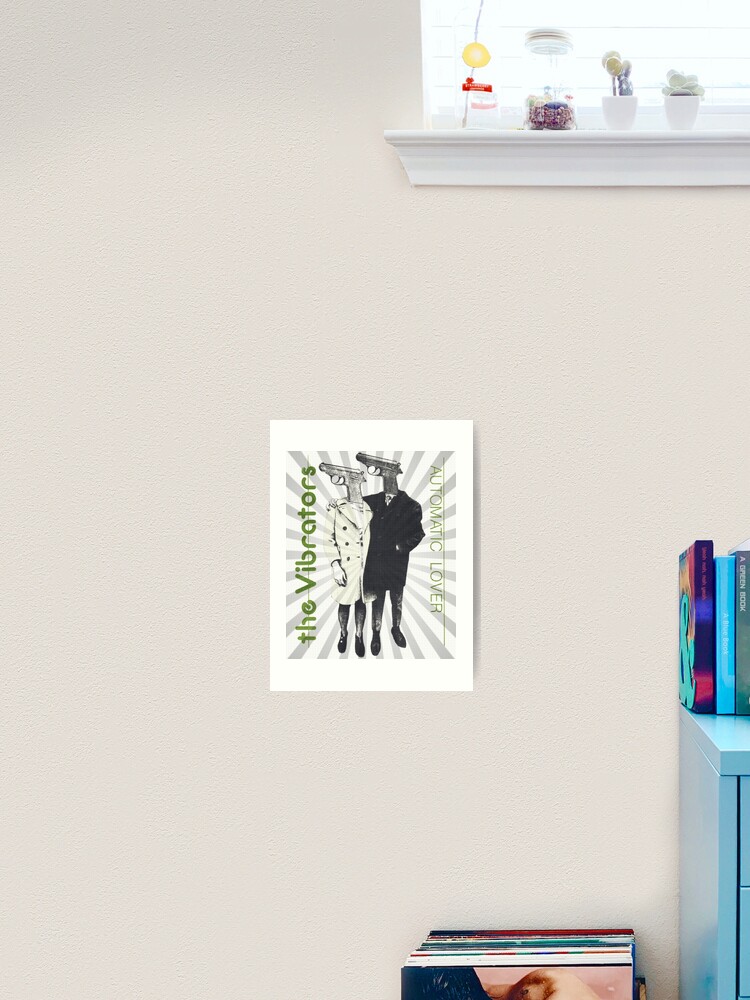The photograph portrays an indoor scene dominated by a light gray wall. Centrally displayed on the wall is a rectangular poster resembling an album cover, featuring a surreal drawing of two figures dressed in contrasting trench coats—one white and one black—with handguns in place of heads. The poster is titled "The Vibrators" written vertically in green on the left side, and "Automatic Lover" in the same fashion on the right, against a backdrop of gray and white lines. In the top right corner of the image, a window allows daylight to stream in, illuminating a windowsill adorned with several glass jars and small potted plants, including miniature cacti. The bottom right corner reveals a partially visible blue cabinet with several books on top, and nearby on the floor, the top edges of some vinyl record sleeves can be seen.